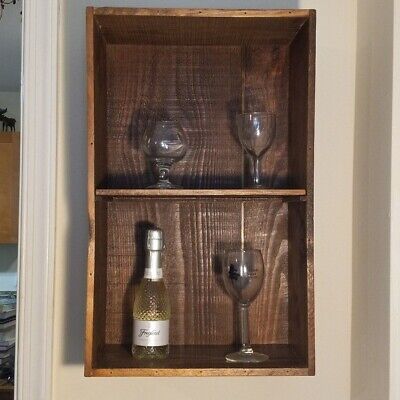The image features a rustic wooden shelf mounted on a cream-colored kitchen wall. The shelf has an open, cabinet-style design with a rich wood grain that gives it a warm, inviting feel. It consists of two shelves: the top shelf showcases two mismatched wine glasses – one tall champagne flute and one shorter goblet, while the bottom shelf holds a standing bottle of unopened white wine next to another uniquely designed wine glass. The backdrop includes a noticeable gray shadow on the right side, adding subtle contrast to the overall scene.